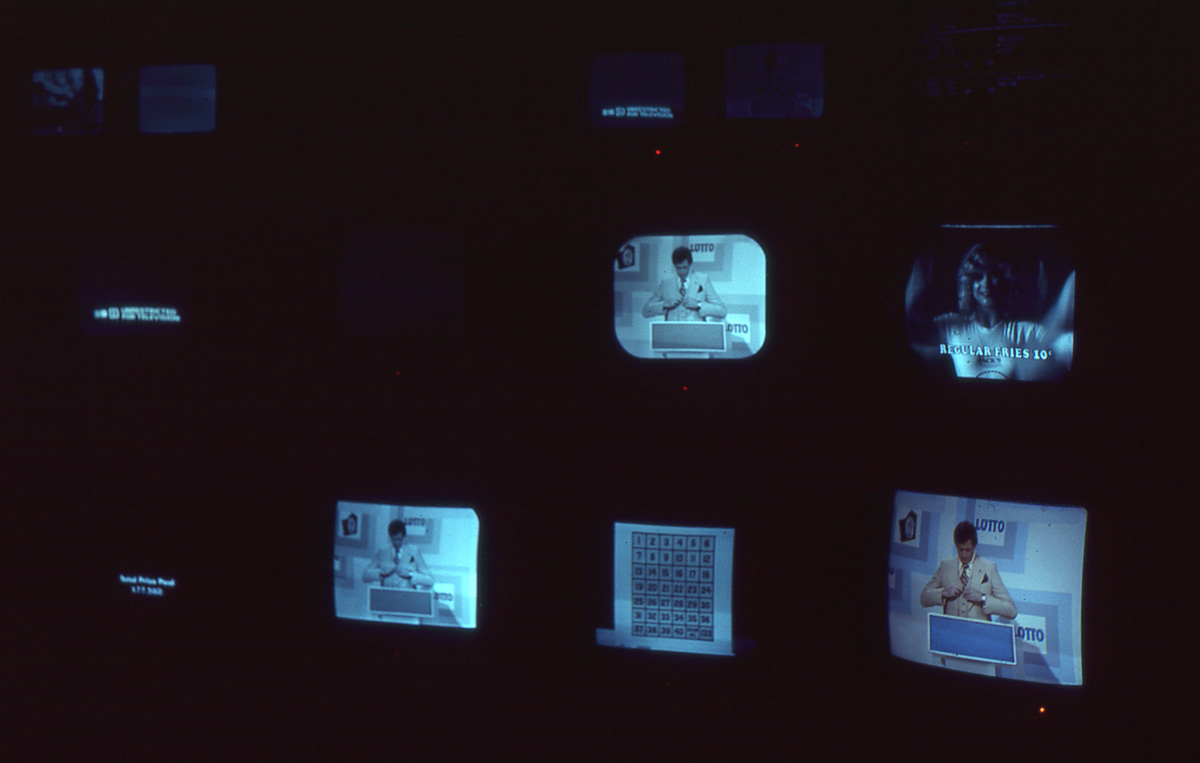In this dimly lit photograph, a collection of older, square TV screens is set against a pitch-black background. The TVs are arranged in a loose triangular formation, with three prominent screens forming the vertices: one on the left, one on the top right, and one on the bottom right. The bottom right screen is more vividly colored, showcasing a man in a tan suit, adjusting his tie while standing at a podium with a blue square and the word "Lotto" inscribed in blue text within a white square below him. This same image repeats on the middle left and middle right screens.

The top right TV screen features a woman with curly hair wearing a white shirt, accompanied by the text "Regular fries, 10 cent." In the center of the formation, another TV screen displays a grid of numbers. The far-left portion of the photograph reveals two additional TV screens stacked vertically, but the content is mostly obscured, showing only some faint blue text. The overall scene is steeped in darkness, creating an almost surreal contrast with the illuminated screens, which remain the primary focus amidst the shadowy backdrop.